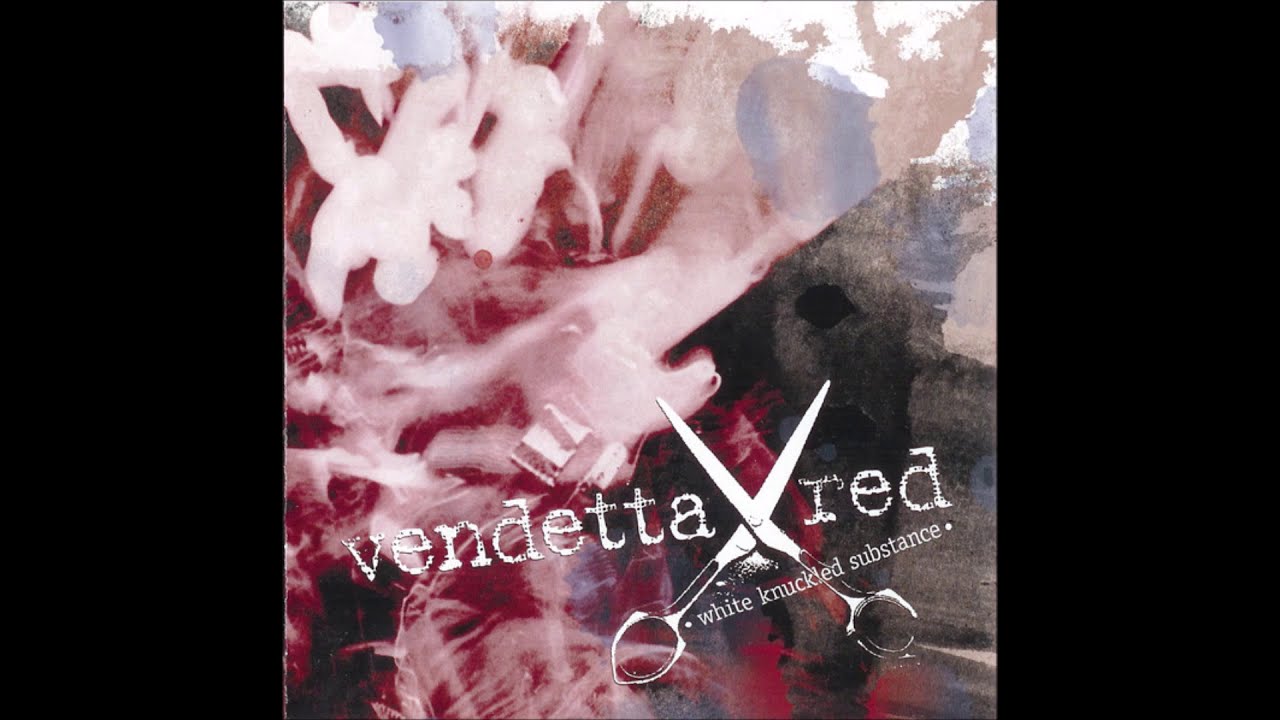The image is a rectangular, landscape-oriented photograph that could be an album cover, advertisement, or brochure. It features two vertical black bars, each about an inch and a half wide, running along the left and right edges. In the center, there is a four-inch by four-inch square picture showcasing a layered abstract design with colors like white, light blue, charcoal gray, red, peach, and pink, giving it a hazy, smoky, or watercolor effect.

At the bottom of the image, angled slightly to the left, is the band name "Vendetta Red" written in a white typewriter-like font, lightly speckled with black spots. Between the words "Vendetta" and "Red," there's an open pair of white computer-generated scissors, creating a 'V' shape. Over the finger holes of the scissors, the text "White Knuckled Substance" appears in a smaller serif font. The total dimensions of the image are approximately six to eight inches wide by five inches tall.